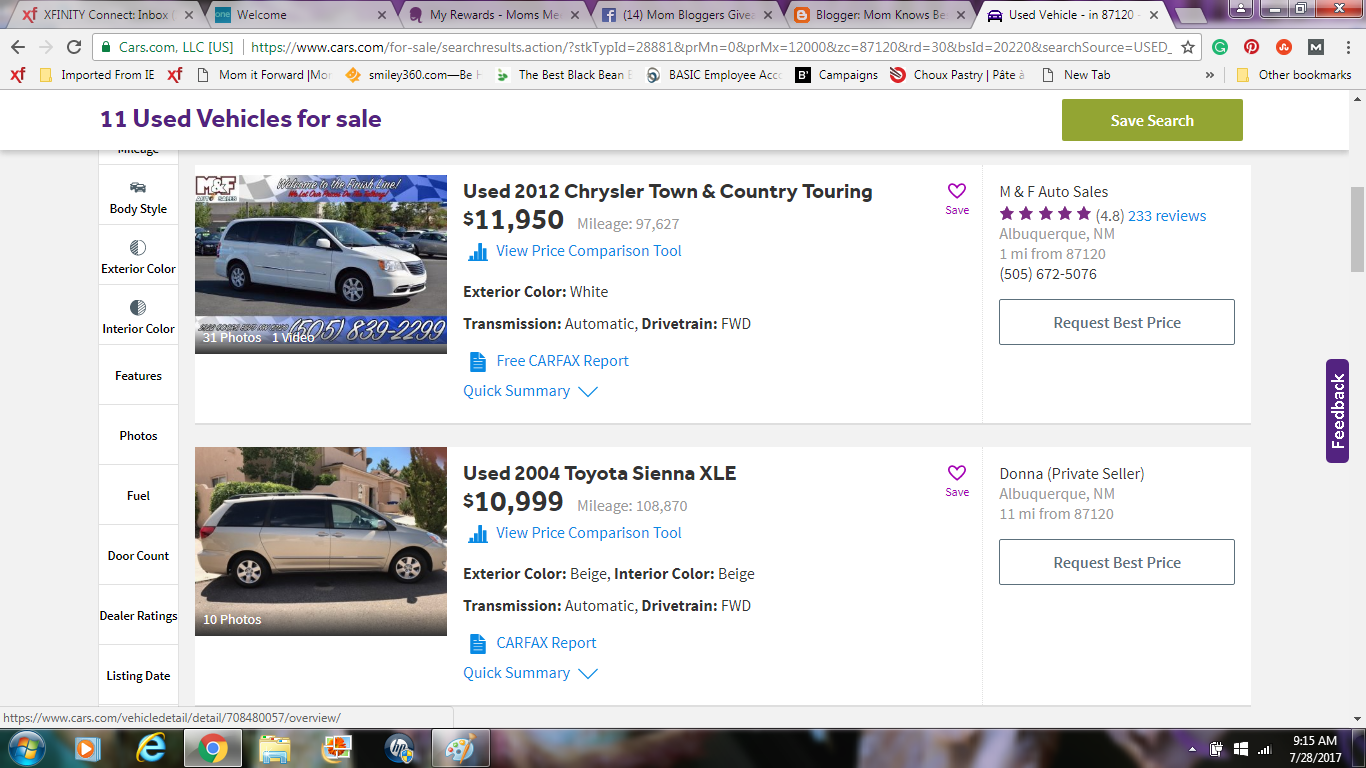A person is using their laptop to browse a used car marketplace on the website cars.com, LLC. The browser shows multiple open tabs, including "Infinity Connect," "Welcome," "My Rewards," "Mom Blogger," "Mom Knows Best," and "Used Vehicles." The current tab, "Used Vehicles," displays a listing of 11 used cars for sale, with images and details for two specific vehicles.

The first vehicle is a 2012 Chrysler Town and Country Touring priced at $11,950 with 97,627 miles. Key features include a white exterior, automatic transmission, and details indicating it's a wheel drive vehicle. Buttons for viewing the price comparison tool and obtaining a free CarFax report are prominently highlighted in blue. The quick summary is also available. The dealership, M&F Auto Sales, provides their location and contact number, with an option to request the best price in a highlighted box.

Next to it, the details of a 2004 Toyota Sienna XLE are listed. It is priced at $10,999 with a mileage of 108,870. The exterior is beige with matching beige interior, automatic transmission, and a front-wheel drive (FWD) drivetrain. Similar options for viewing the price comparison tool and accessing the CarFax report are available in blue links, along with a quick summary.

On the left side of the listings, categories such as exterior color, interior color, features, photos, fuel type, door count, dealer ratings, and listing date are outlined. At the bottom of the screen, there's a faint image, though it's too blurry to make out any details.